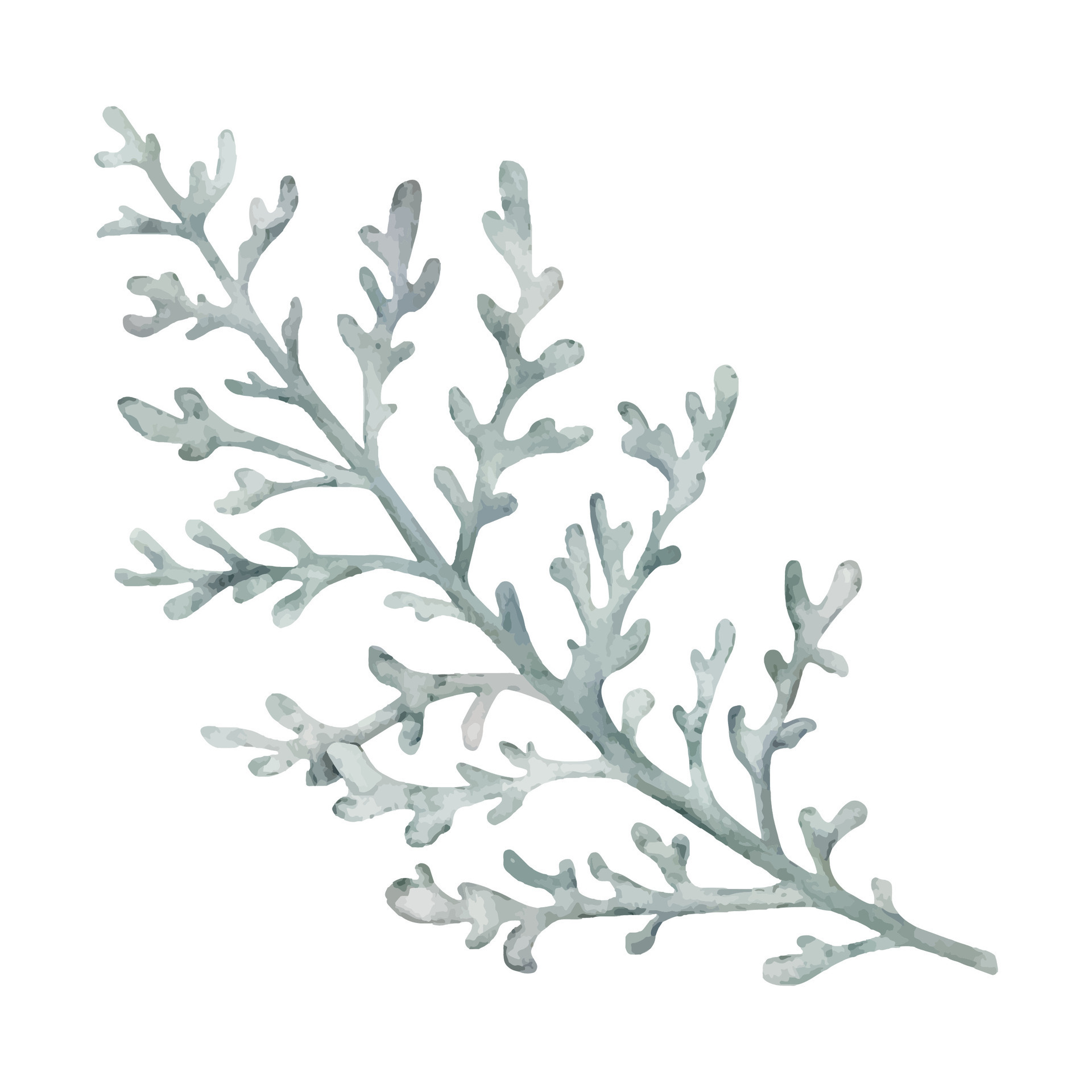This illustration features a stylized, watercolor-like painting of a plant stem, depicted in a light greenish-gray to light forest green color palette against a crisp white backdrop. The central stem rises diagonally from the bottom right to the top left corner of the image. Branches extend from the central stem in a pattern that resembles antlers, creating a series of V-shaped formations on either side. Each primary branch further divides into multiple smaller branches, all terminating in rounded tips. Some of these smaller branches bear clusters of leaves, with certain clusters containing two, three, four, and even up to ten leaves. The overall texture and style of the portrayal give it an artistic, non-lifelike appearance, yet the intricate detailing of the branching structure and leaf arrangements adds a sense of natural complexity and beauty.